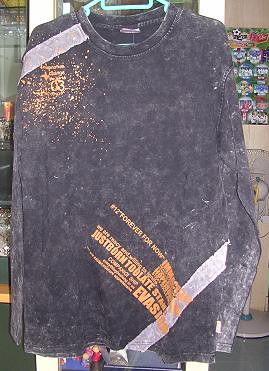This photograph captures a grungy, worn, long-sleeved black sweatshirt hanging on a light teal plastic hanger. The sweatshirt features a distinctive design with white diagonal stripes located on the right shoulder and bottom left area. Scattered orange speckles adorn the upper left shoulder area, adding to its grungy aesthetic. The somewhat faded and hard-to-read orange text is strategically placed, with some text on the right shoulder corner and more text running diagonally across the lower abdomen area. The visible words include "12thforeverfornow," "just born too late," "evasion," and possibly other random words, contributing to its edgy, urban appearance. The overall look and the staging suggest that this photograph may be intended for an online sale platform, potentially showcasing the apparel in a store-like environment.